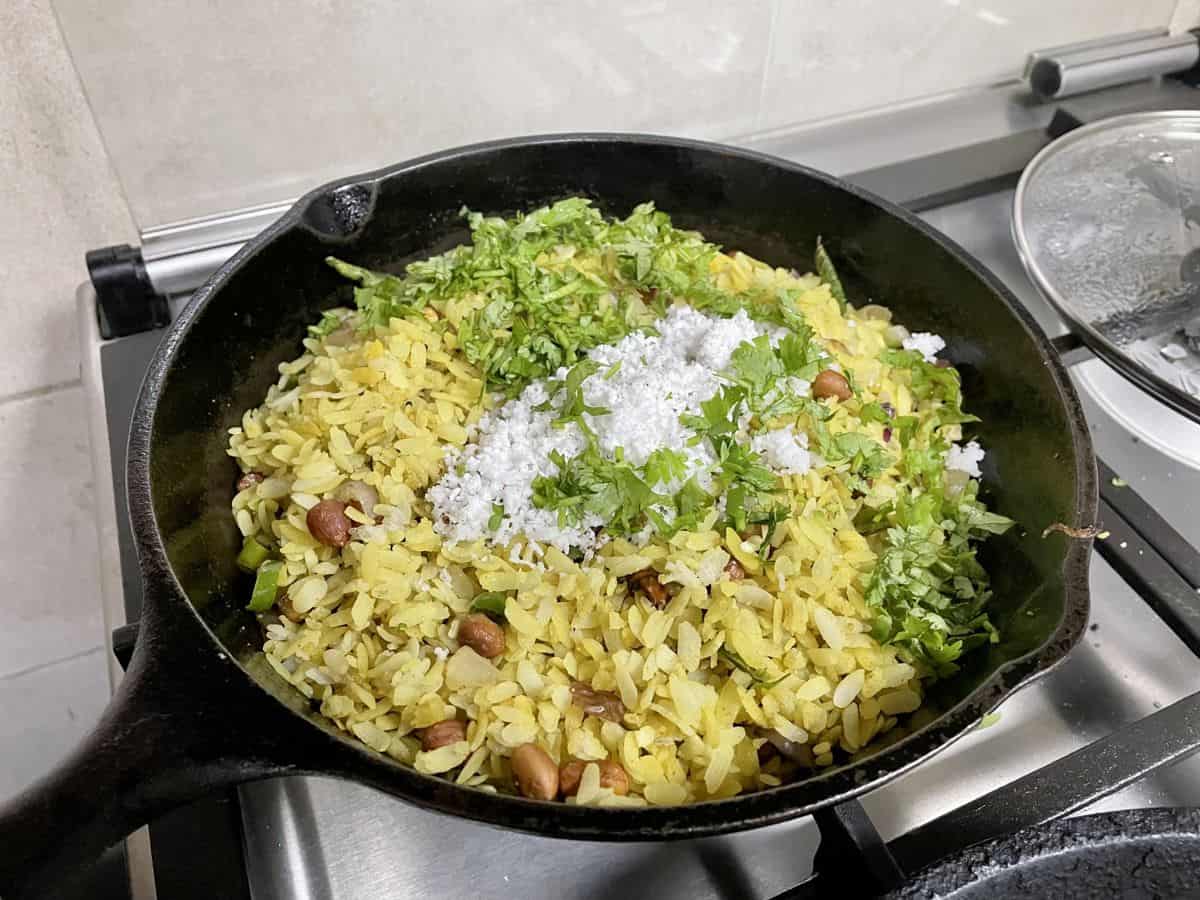The image features an old and worn 10-inch black cast iron skillet situated on a gas range. The skillet contains a mix of large yellow grains that resemble rice, interspersed with brown beans, possibly pinto beans, and green elements that could be broccoli or parsley sprigs. In the center of the pan is a notable pile of finely grated white substance, which might be Parmesan cheese. Adjacent to the skillet, on the burner, is a glass lid with visible steam on the inside, indicating it was recently removed from the pan. The stove top and surrounding area show a glimpse of another cast iron pan's handle towards the bottom right, and white tile surfaces are visible on the left side of the image.